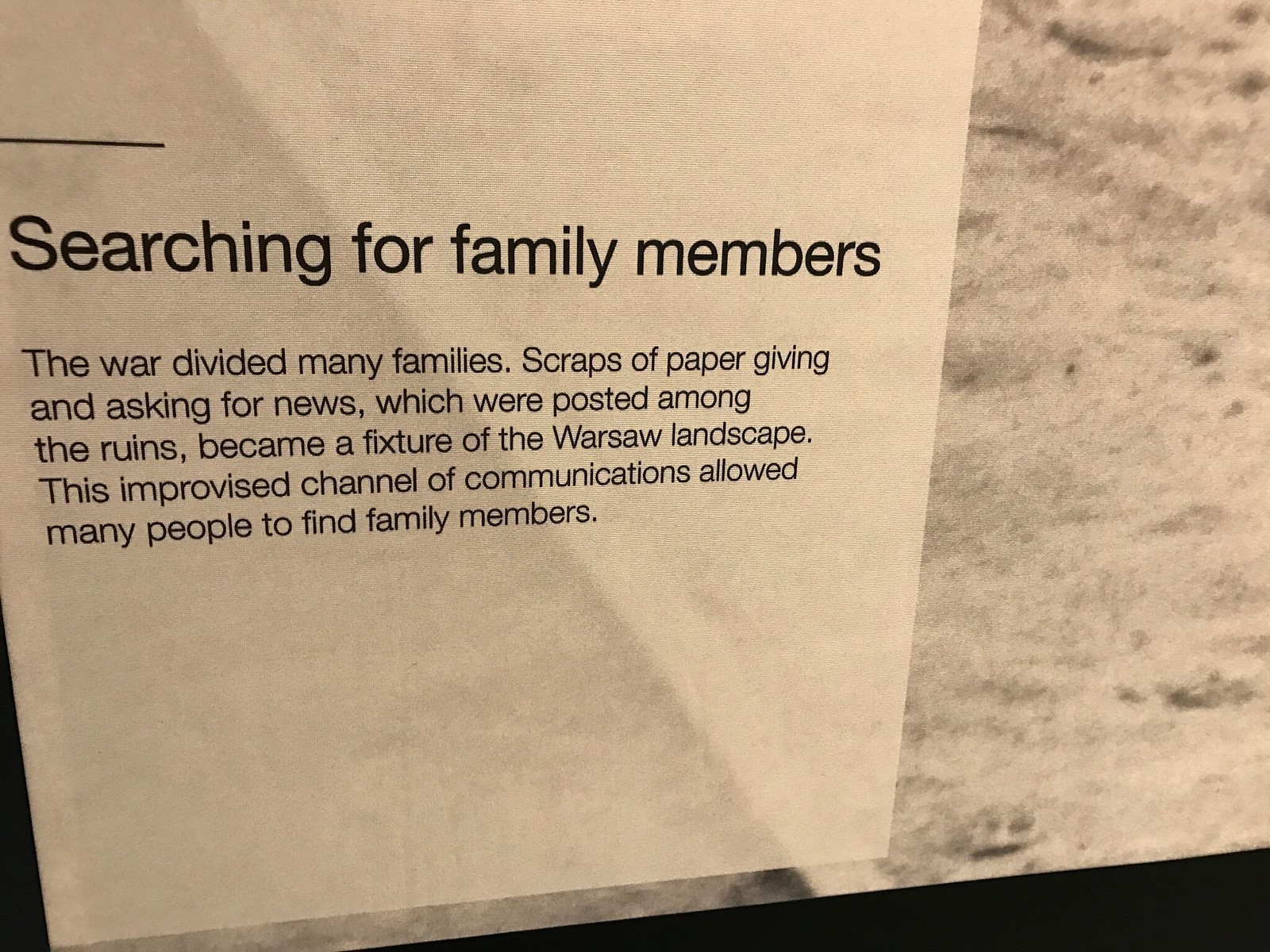The image displays a museum exhibit titled "Searching for Family Members." It features a sign with the text: "The war divided many families. Scraps of paper giving and asking for news, which were posted among the ruins, became a fixture of the Warsaw landscape. This improvised channel of communications allowed many people to find family members." The sign is cream-colored with black text and is centrally positioned within the photograph. Behind the sign, a sandy soil surface is visible, adding to the historical ambiance. This display poignantly illustrates how wartime communications through posted scraps of paper helped reconnect separated families in Warsaw, evoking memories of the war's impact on families and the city's landscape. The exhibit's detailed presentation emphasizes the significance of these messages in the collective memory of the community.